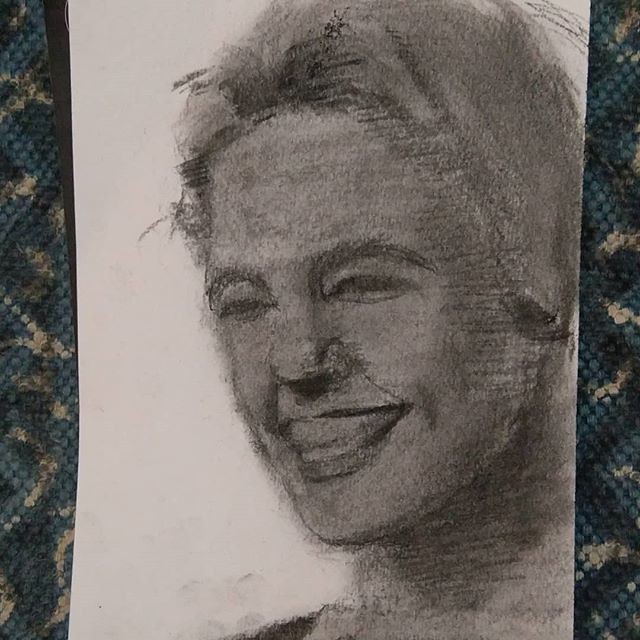The image features a detailed charcoal or pencil headshot drawing of a smiling woman with short or pulled-back blonde hair. Her squinty eyes and visible teeth highlight her cheerful expression, though her pupils and exact gaze direction are indiscernible due to the dark shading. The sketch is centered on an off-white sheet of paper and captures her face and shoulders, extending to her collarbone. The paper is set against a textured, haphazardly patterned background reminiscent of thick Mexican blankets with circular fabric beads. This background consists of black, teal, and off-white colors, letterboxing both the left and right sides of the image by approximately 15%, creating a striking contrast to the monochromatic drawing. The woman, positioned slightly to the right and angling her face towards seven o'clock, exudes a sense of warmth and attractiveness despite the blurred details.